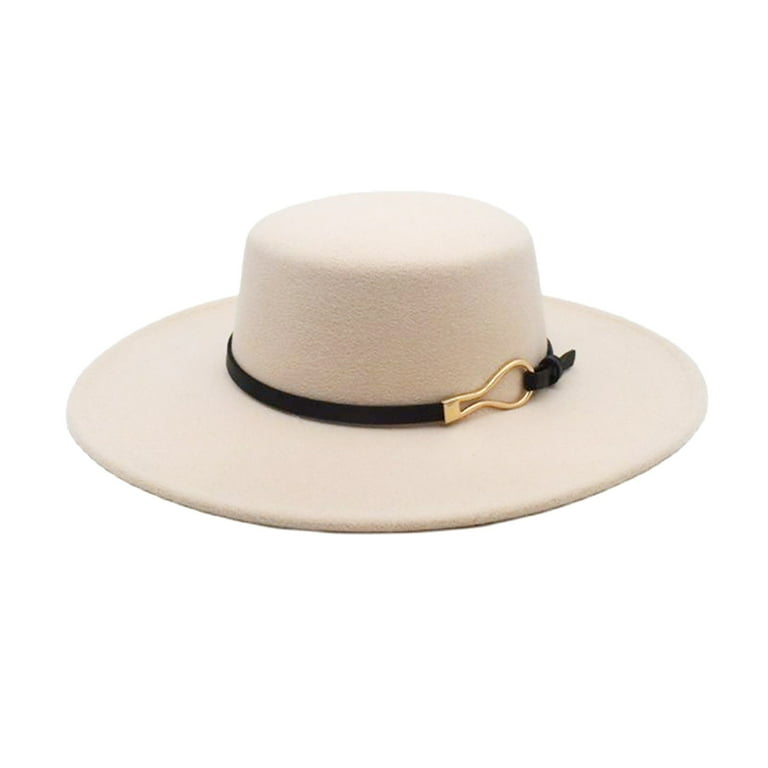In the center of this image is a wide-brimmed hat, primarily light beige or cream in color. The hat features a flat top and a straight, round brim designed to block sunlight. Around the middle part of the hat, there is a thin black band-like strap, which is fastened by a gold loop, adding a touch of elegance. The background of the image is solid white, ensuring that the details of the hat stand out prominently.